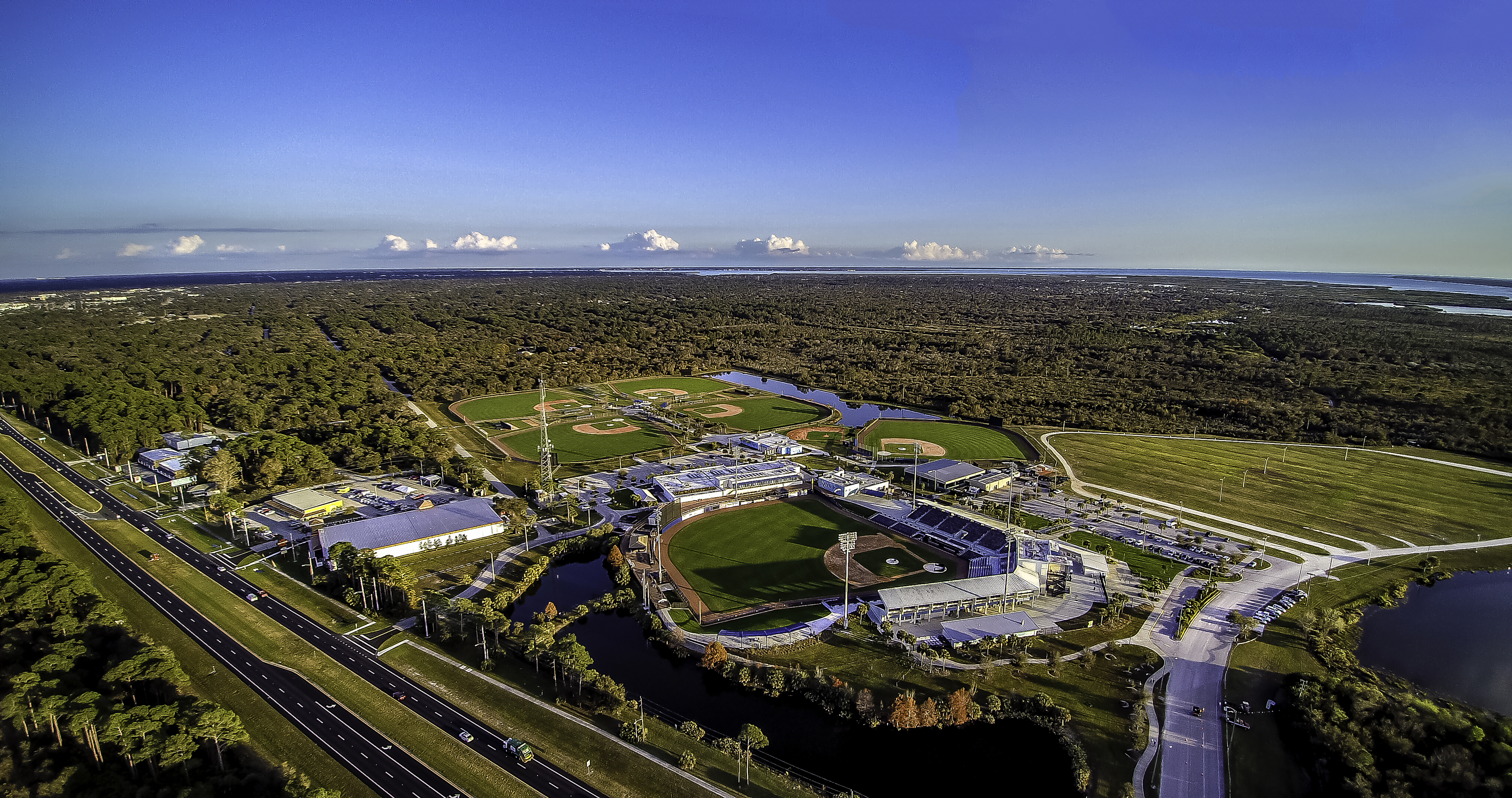This aerial photograph captures a sprawling sports complex featuring six neatly manicured baseball fields encircled by lush green trees. The image, likely taken by a drone or aircraft, reveals a large, well-maintained stadium with ample seating capacity. Surrounding the stadium are additional baseball diamonds, all appearing clean and well-kept. Adjacent to the fields, there are several white buildings and bleachers for spectators. A significant highway runs next to the complex, with sporadic traffic indicating a typical daytime scene. In the background, a serene landscape unfolds with patches of forest and a picturesque lake to the right. Further in the distance, another smaller body of water is visible near the fields, with wispy clouds scattered across a brilliant blue sky. Additionally, a large parking lot accommodates visitors to this bustling hub of athletic activity.